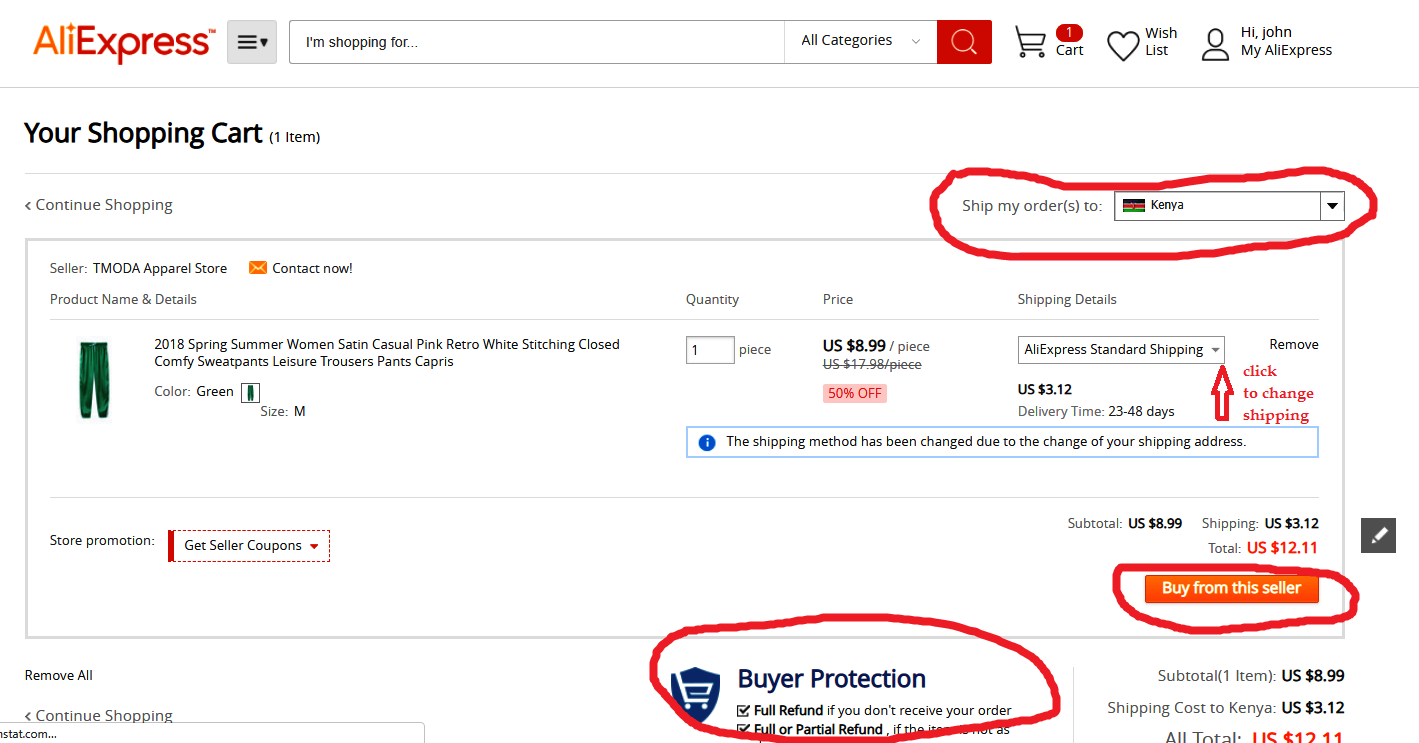This is a screenshot from the AliExpress website. In the top left corner, the words "AliExpress" are displayed with "Ali" in orange and "Express" in red. Adjacent to this is a gray square containing three horizontal black lines and a downward-pointing arrow. Next to the gray square is a search bar with black font that reads "I'm searching for..." At the end of the search bar, there is a drop-down menu labeled "All Categories" followed by a red square featuring a white magnifying glass icon, indicating the search function.

To the right of the search bar is a black shopping cart icon with the word "Cart" next to it, along with a red badge above it showing the number one, indicating there is one item in the cart. Further to the right, there is a heart icon labeled "Wish List," followed by a silhouette of a human figure accompanied by the text "Hi John, my AliExpress."

Below this top section is a black horizontal line, under which the text "Your shopping cart 1 item" appears. Another black horizontal line separates this from the text "Continue Shopping" accompanied by a left-pointing arrow on the left side, and the text "Ship my orders to" on the right side, which has been circled in red using a paint program. Next to this, a box indicates "Kenya" as the shipping destination. Below this section is a black-outlined rectangle displaying the item to be shipped, which is a pair of pants.